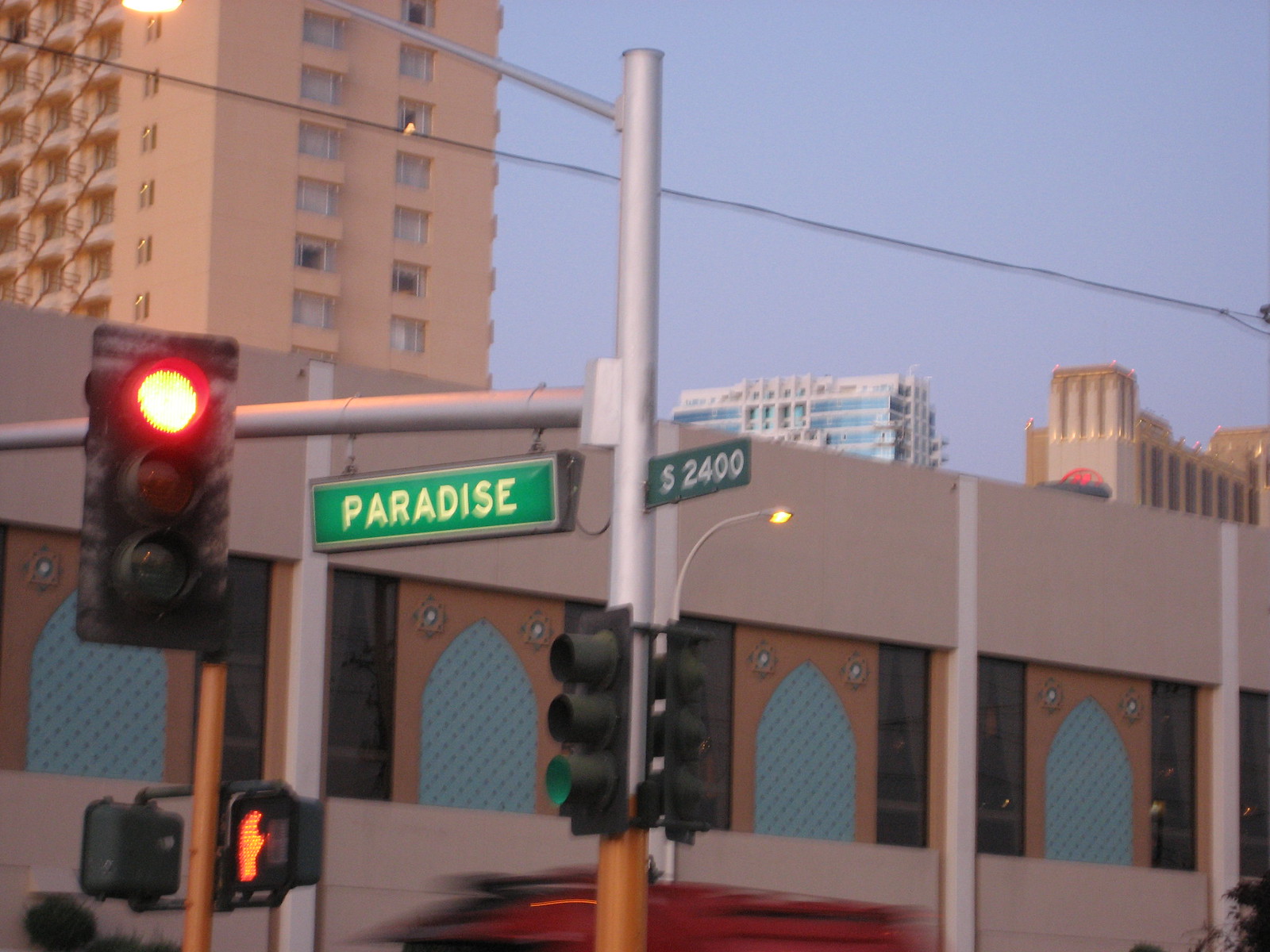This photograph, seemingly taken from a city street, showcases a scene under a dull bluish-gray sky. The sky appears to be hazy, possibly due to overcast conditions or the lighting affecting the photograph. The backdrop features a tall apartment building with striking red walls and an array of rectangular windows, suggesting a residential complex. Flanking this structure, further in the distance, are other tall edifices that could either be hotels or more apartment buildings.

In the foreground, the upper edge of a shorter commercial building is visible, characterized by white panels and faux arched windows. Dominating the scene is a streetlight pole, appearing newly brushed and metallic, with various street signs attached. One sign prominently reads "Paradise" in white letters on a green background, while another sign indicates "S-2400," likely referring to a street location or directional marker.

Attached to the pole are traffic lights and a pedestrian walk signal. The traffic light facing the camera shows a red light, while the light oriented in the opposite direction is green. Additionally, the crosswalk signal displays a red hand, indicating pedestrians should not cross. The overall impression of the environment, combined with the architectural elements and the street signage, suggests a bustling urban area, possibly situated in a warmer climate based on the light-colored beige buildings and the overall atmosphere.